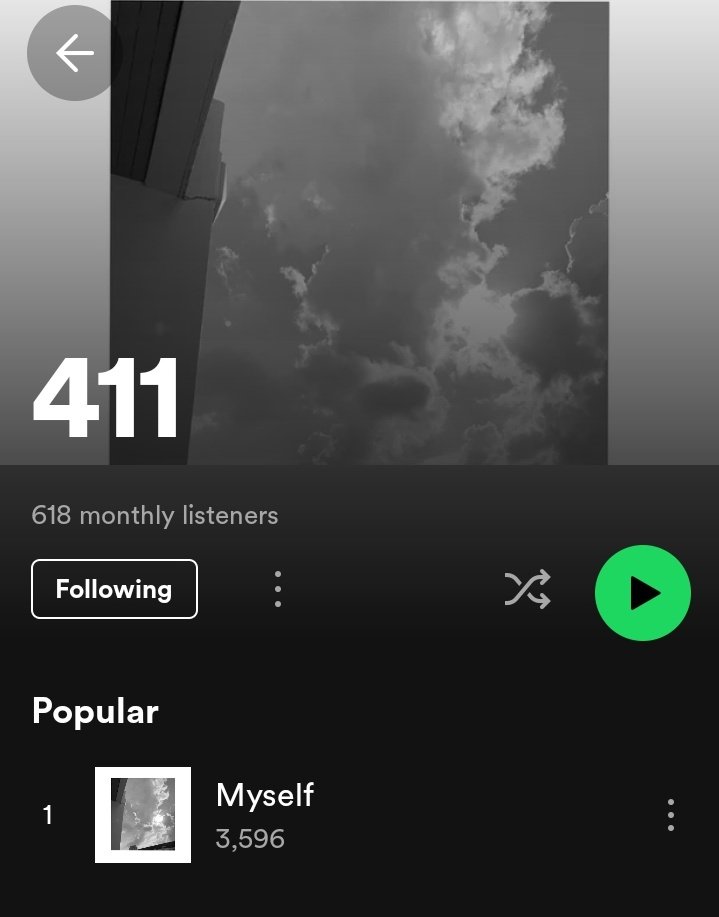This screenshot from a Spotify artist page showcases a monochromatic aesthetic centered around a grayscale photograph of a cloudy sky. On the left half of the photo, the edge of a building or its façade is partially visible, while on the right, a luminous orb—likely the Sun or the moon—is surrounded by dense clouds with gray centers and wispy, white edges.

In the bottom-left corner of the photo, bold white text displays the string "411." The upper left corner features a gray circular button with a white arrow pointing left, suggesting a navigation option. Below the main image, the text "618 monthly listeners" appears on a black background.

A white-outlined rectangle with the word "following" in white text is present below the listener count, accompanied by a gray ellipsis button and a gray shuffle icon. Adjacent to these is a large circular green button with a black play triangle in its center, indicating the play feature.

Further down, bold white text labels the section "Popular." Under this heading, a small thumbnail of the previously described cloudy sky scene is next to the number one, with the song title "myself" and the play count "3,596" in white text. A gray ellipsis button sits to the right of the song details, providing additional options.